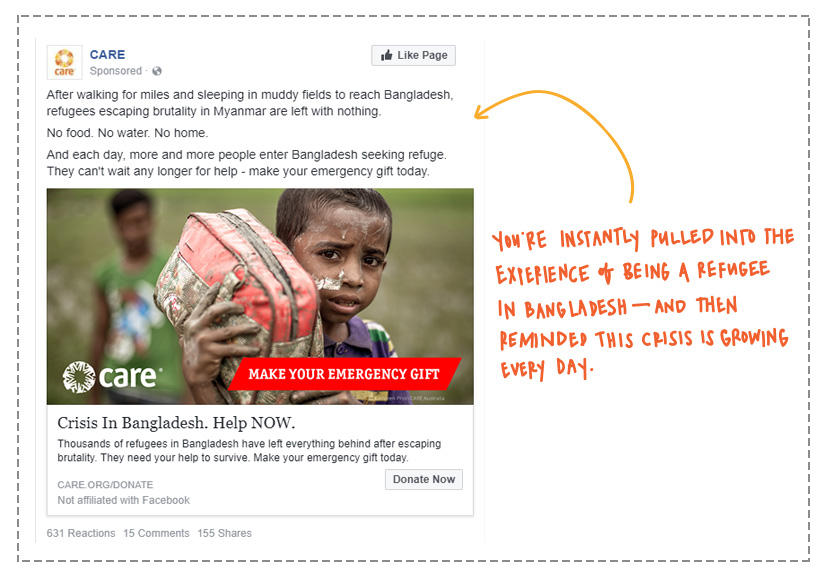This poignant image is a heart-wrenching portrayal of the dire situation faced by refugees who have fled from Myanmar to Bangladesh. The logo of Care, a humanitarian organization, is prominently displayed in the upper left corner, featuring a white box with the word "Care" written in bold red letters and a yellow circle beside it. Below the logo, the word "Sponsored" is indicated, and a small box with a thumbs-up icon invites viewers to "Like Page."

The border of the webpage is adorned with a pattern of dotted gray lines, giving a sense of continuity and framing the content. The emotional appeal is accentuated by a moving narrative: "After walking for miles and sleeping in muddy fields to reach Bangladesh, refugees escaping brutal persecution in Myanmar are left with nothing—no food, no water, no home. Each day, more and more people seek refuge in Bangladesh. They can't wait any longer for help. Make your emergency gift today."

The central image captures a young boy, his face and clothes smeared with mud, holding a bag over his shoulder. His expression is one of deep contemplation and intensity. A figure behind him, possibly a family member, is visible wearing a green t-shirt and sporting brown hair. 

Highlighted in red across the bottom of the boy's body are the words "Make your emergency gift today." To further illustrate the urgency, the text next to the image reads, "You're instantly pulled into the experience of being a refugee in Bangladesh. This crisis is growing every day." A yellow arrow points to the phrase, "Crisis in Bangladesh: Help now," emphasizing the critical need for aid.

The page also includes a call to action: "Thousands of refugees in Bangladesh have left everything behind after escaping brutality. They need your help to survive. Make your emergency gift today," followed by a prominent "Donate Now" button. At the bottom, it is noted that "Care is not affiliated with Facebook," and options for reactions and comments are available.

The entire presentation is a powerful and urgent plea for immediate assistance to support the countless refugees in desperate need.